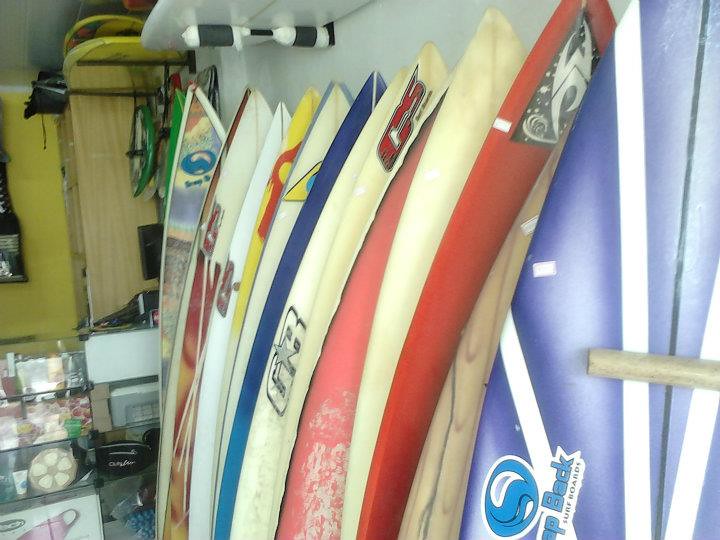This image captures the interior of a surf shop, where approximately ten colorful surfboards are prominently displayed. The surfboards are stacked upright, leaning against a yellow wall in the foreground, directly beneath a white shelf. These boards feature a variety of colors including purple, blue, red, white, tan, yellow, and pink. Notably, the nearest surfboard is purple and white with the partially visible words "Back Softboard" on a sticker. Other boards exhibit diverse patterns such as a wood grain design, a red slash, a flame pattern, and even a cityscape image.

In the background, the shop features wooden cabinets and glass display cases showcasing various surfing accessories, likely surfboard wax and other related items. Off to the right, there appears to be the checkout counter with additional merchandise. The overall setting strongly indicates an indoor surf shop, with the vibrant surfboards and well-organized displays forming the core focus of the space.